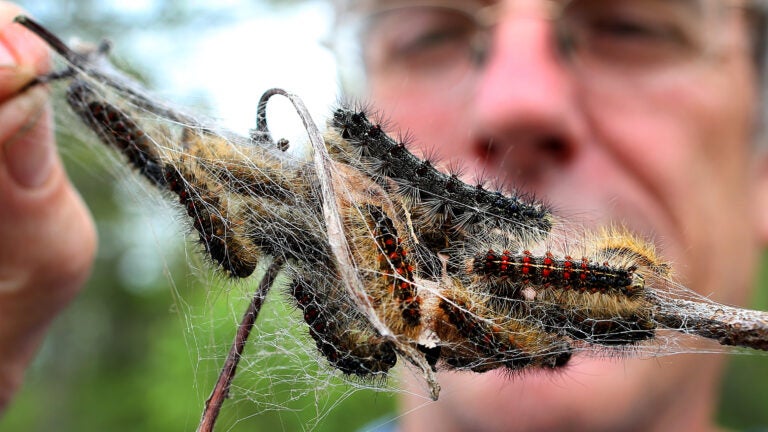In this close-up image, a man wearing glasses and slightly out of focus is standing behind a stick teeming with at least a dozen caterpillars. The man, who appears to be older judging by the wrinkles on his face, is carefully holding the stick and observing the caterpillars, which are the main focus of the image. The stick is enmeshed in a web-like silk structure, indicating it may have been a nest for the caterpillars. The caterpillars themselves are quite hairy, with a mix of black, red, and gold hairs. While most of them are similar in size, they display a variety of colors, including some that are yellowish and some black with red spots. The background of the image shows green trees, suggesting an outdoor setting. The caterpillars' intricate silk webbing and their diverse appearances create a visually intriguing scene.